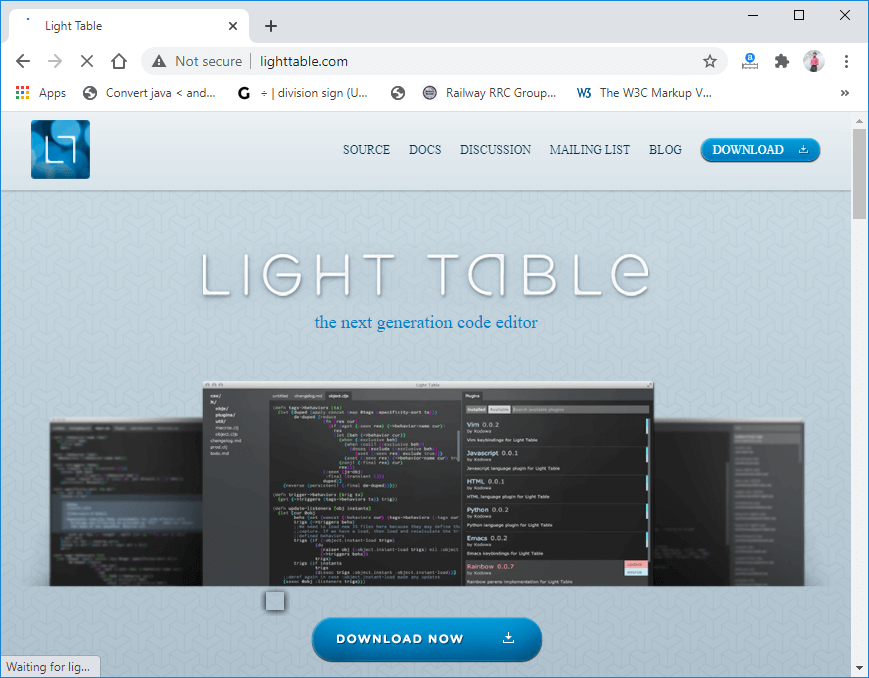The image is a screenshot of a browser window, likely Google Chrome, displaying the Lighttable website. The browser is open to the Lighttable landing page, showcasing its sleek user interface. In the upper left corner of the page, there's a small graphic featuring a stylized "L" and "T" with a bokeh effect background.

At the top navigation bar, there are several links labeled Source, Docs, Discussion, Mailing List, Blog, and a prominent Download button. Below this navigation bar, the main content area introduces Lighttable as "the next generation code editor." 

The central part of the landing page features an image showcasing a series of command line interface windows with code displayed. The code within these windows is indistinct due to the resolution of the screenshot, but the presence of multiple open windows highlights the product’s capability of managing several code workspaces simultaneously.

Towards the bottom of this section, there is a large blue button labeled "Download Now" accompanied by a download icon, encouraging users to obtain the software.

Finally, at the very bottom of the screen, a message partially reads "Waiting for lig...", suggesting that the page is still loading further content. On the far right side, a scroll bar indicates that additional information is available by scrolling down the page, likely providing more details about Lighttable's features and benefits.